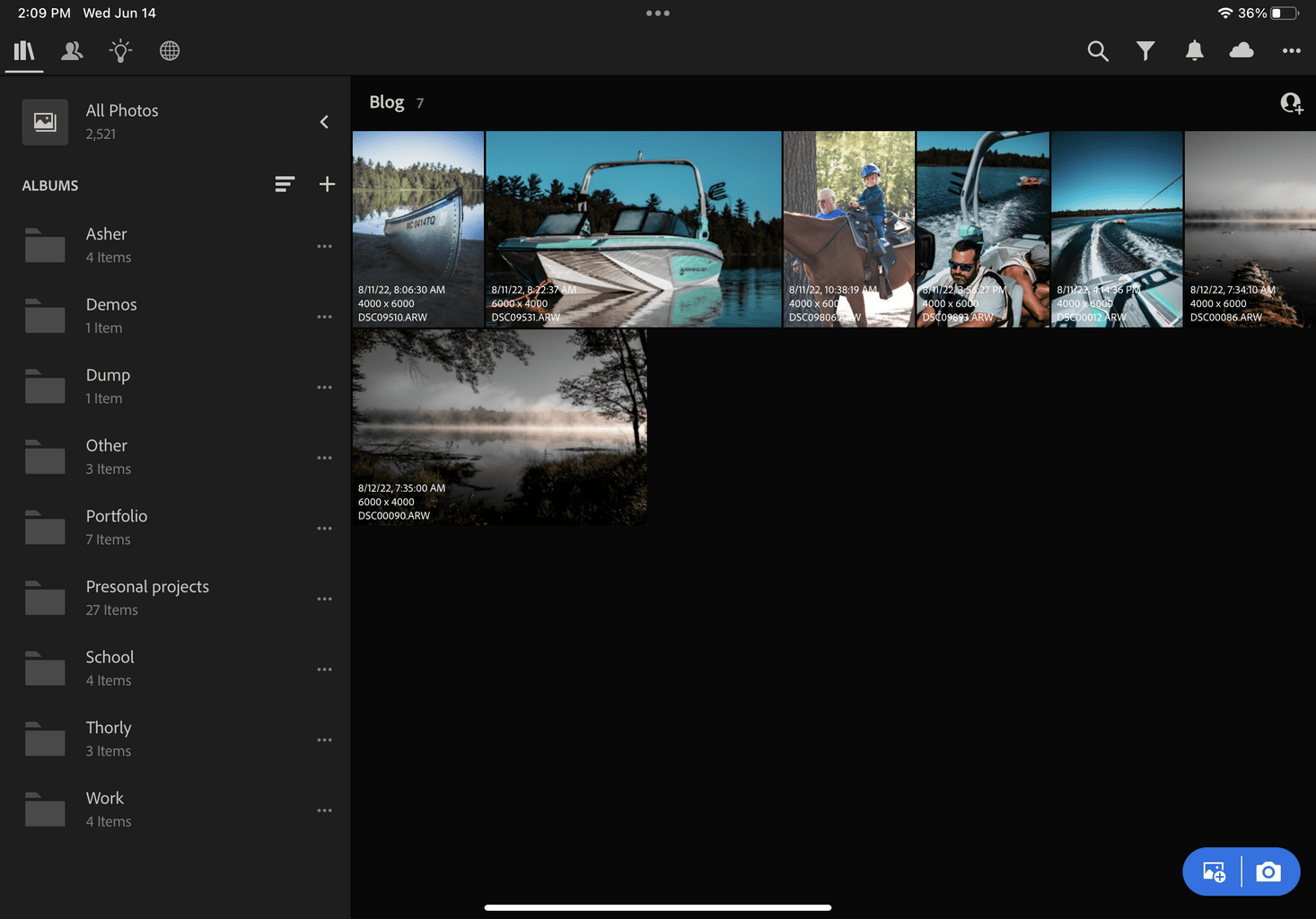This image, captured from a computer screen, showcases an online photo album interface with a black background. The aspect ratio is wider than it is tall, confirming it as a desktop view rather than a mobile one. 

In the upper left corner, a timestamp reads "2:09 PM, Wednesday, June 14th" without specifying the year. Below the timestamp, four icons are displayed, with the leftmost one, resembling a series of books, highlighted by a horizontal gray line — it represents photo albums.

On the upper right corner, various system icons are visible, including search, notifications, and cloud storage. The battery indicator shows a 36% charge, while data connectivity appears to be strong.

The left-hand column of the interface lists the categorization of photos, starting with a total count of 2,521 under the "All Photos" section. These are further organized into albums labeled Asher, Demos, Dump, Other, Portfolio, Personal Projects, School, Thorley (spelled T-H-O-R-L-Y), and Work.

The main screen prominently features a "Blog" section against the consistent black background. Six photographs are aligned at the top with one more positioned at the bottom. Each photo carries timestamps, like "8, 11, 22," indicating they were taken two years ago. The top row primarily contains images of boats on a lake, with one exception — a photograph of horses.